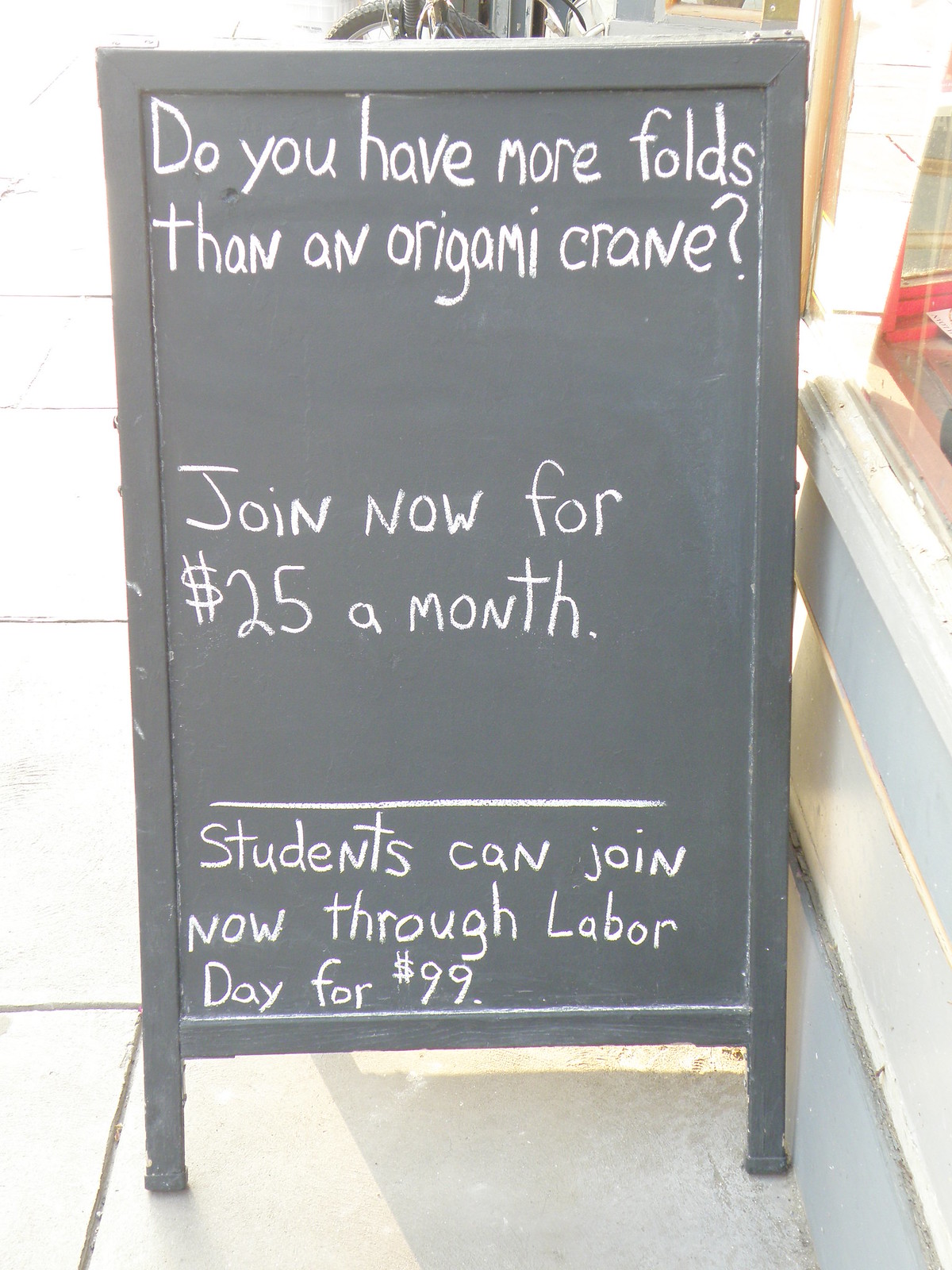This image captures a promotional blackboard sign positioned outdoors on a stone pavement walkway, presenting a striking advertisement for a potential gym membership. The blackboard, with its chalk-written text in white and accents of pink, boldly questions passersby, "Do you have more folds than an origami crane?" Beneath this playful query, it invites individuals to "Join now for $25 a month," followed by a horizontal dividing line and an additional offer stating, "Students can join now through Labor Day for $99."

The setting's ambiance is enhanced by the surrounding environment: the sign is flanked to the right by a white-walled building that includes a partially visible window, through which a glimpse of a red object can be seen. Directly behind the sign, faint outlines of a bicycle wheel peek through. With an overall bright lighting indicative of daytime, the photograph highlights the sign's functional design, resting on skinny supporting legs against the tan concrete tiles. This evocative scene suggests a casual yet engaging outdoor advertisement for a local gym.